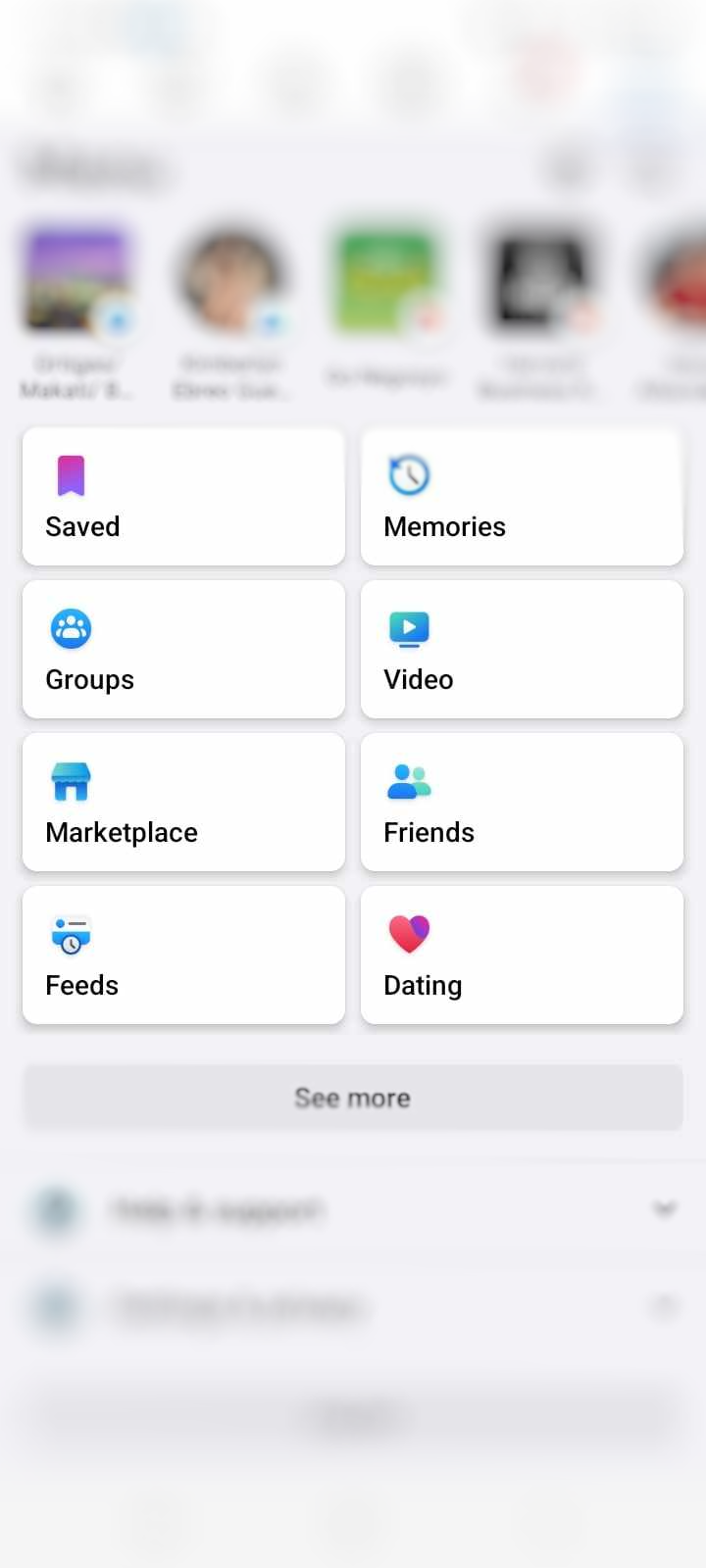This is a detailed screenshot captured on a mobile phone displaying a user's Facebook app interface. The top portion of the screen has been deliberately blurred to obscure certain personal details such as the list of followed individuals, recent story posts, and interactions with friends or family linked via Instagram. However, the visible portion of the screen reveals several navigational sections including 'Saved Posts,' showcasing posts the user has saved, 'Memories,' highlighting past activities and posts, and 'Groups,' indicating communities the user is part of or interested in. Additional features include access to 'Videos,' showcasing available video content, and the 'Facebook Marketplace,' which is identified by a blue hut icon and labeled "Marketplace," allowing the user to browse and shop items. There are also sections for 'Friends,' providing access to the user's friend list, 'Dating,' symbolized by a purple and pink love heart icon, offering dating services, and options for exploring further insights into the user’s history and feed activity.